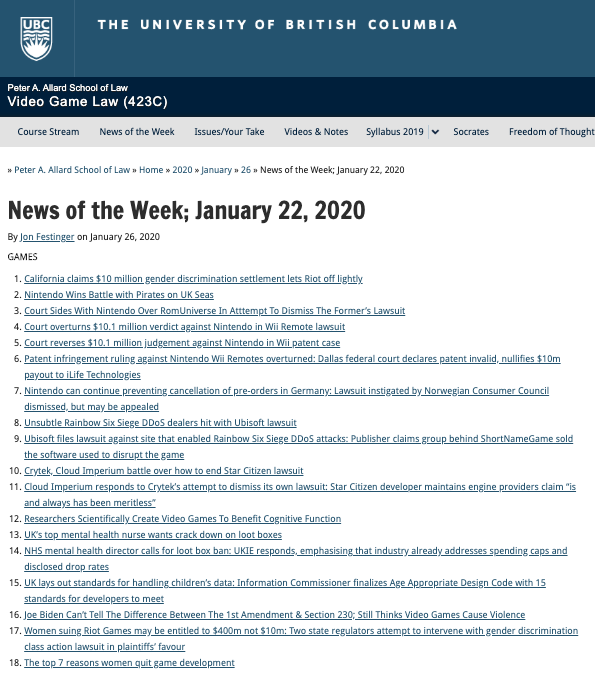The image is a screenshot from an online resource associated with the University of British Columbia. At the top, in a blue header, the university's name is prominently displayed in white text. Adjacent to this is the UBC shield logo, featuring symbols of water and the sun. Below the header, the text identifies the source as the Peter A. Allard School of Law's Video Game Law section.

Centrally positioned in bold black letters, the title reads "News of the Week, January 22nd, 2020" followed by the byline, "by John Festinger on January 26th, 2020." 

The section titled "Games" contains a list of 18 numbered news items written in blue text. The first item highlights a $10 million gender discrimination settlement involving California and Riot Games, stating that the company was let off lightly. The second item details Nintendo's legal victory against game pirates in the United Kingdom. The third news item reports that the court sided with Nintendo in its lawsuit against ROM Universe, successfully dismissing the latter's attempt to quash the complaint.

Further down the list, item number 13 mentions the UK's leading mental health nurse's call for stricter regulations on loot boxes in games. The final news entry, number 18, outlines the top seven reasons women leave the game development industry.